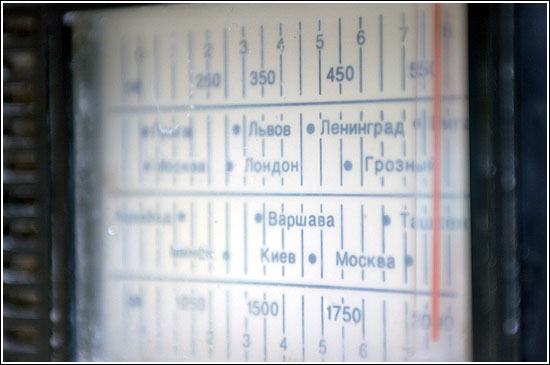The image features a close-up view of a white radio dial, likely from a transistor radio. The dial includes numerical markings in white, enumerating frequencies such as 1500 and 1750, and continues with 250, 350, 450, and so on. Dominating the display is a horizontal red line, which serves as the indicator for tuning into specific stations. This style of radio dial is reminiscent of both AM and FM tuners typically found in desk-sized radios.

Additionally, the dial features an unfamiliar script, including sequences such as "B-A-P-W-A-S-A," which add an enigmatic aspect to the design. Surrounding these peculiar inscriptions are numbers ranging from one to six, positioned both above and below the main frequency markers. It is unclear whether the upper set of numbers corresponds to AM frequencies and the lower set to FM frequencies, or vice versa. The language and formatting present an intriguing and somewhat cryptic appearance that adds to the radio's vintage charm.